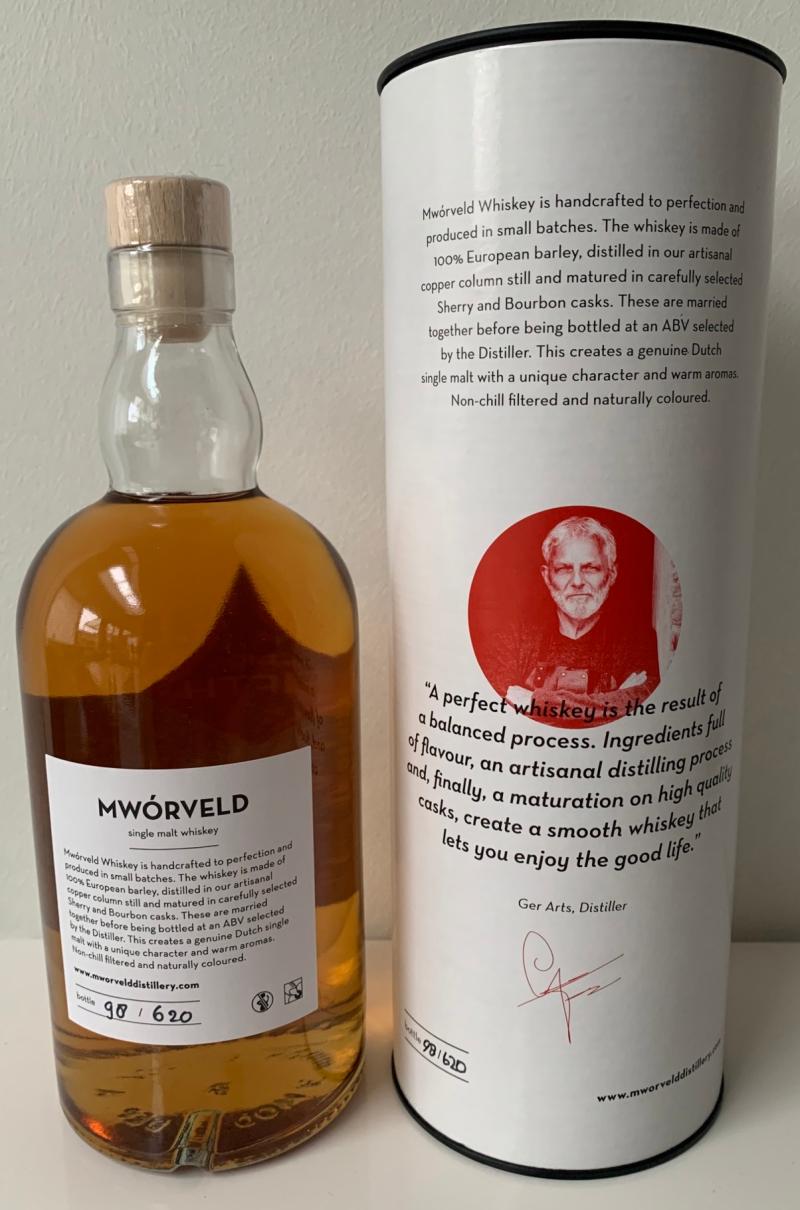This image captures a meticulously arranged display of a handcrafted single malt whiskey named Morveld. The composition features a clear glass bottle filled with golden whiskey, adorned with a light brown cork top, and a detailed label. The whiskey boasts an ABV selected by the distiller, is made of 100% European barley, distilled in artisanal copper column stills, and matured in carefully selected sherry and bourbon casks. The product is described as non-chill filtered and naturally colored, resulting in a whiskey with a unique character and warm aromas. Alongside the bottle stands a white cylindrical container, likely the case for the bottle, which has a black and white photograph of the distiller, Ger Arts, set against a red background. Accompanying the image is a quote that reads: "A perfect whiskey is the result of a balanced process, ingredients full of flavor, an artisanal distilling process, and finally a mature maturation on high-quality casks create a smooth whiskey that lets you enjoy the good life.” The background is a simple white wall and the setup rests on a white table, emphasizing the elegance of the whiskey presentation.